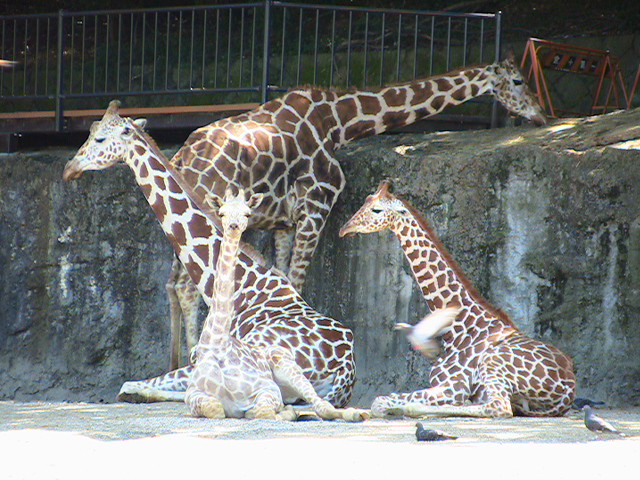This is an outdoor color photograph taken at a zoo, depicting four giraffes within a stone enclosure. The enclosure features a tall, gray stone wall with watermarks and sections of a metal railing on top, partially covered by a red barrier. In the foreground, two smaller giraffes are sitting on a stone or concrete surface. The giraffe on the left is facing towards the camera, appearing to look at the viewer, while the giraffe on the right is facing left. A blurred bird in mid-flight with its wings open is visible in front of this giraffe. Behind them, a larger giraffe is also sitting and looking towards the left. Further back, the largest giraffe stands with its neck stretched out, leaning towards the stone wall, and its head peeking over the top. The giraffes display typical brown and beige coloring, with the adults showing more prominent patterns than the younger ones. Additionally, three pigeons are visible, with two on the ground and one mid-flight, adding a sense of dynamic movement to the scene.